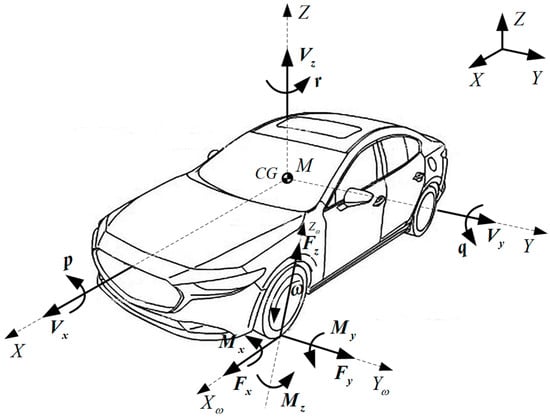This detailed, black and white diagram illustrates a sporty, four-door sedan from a three-dimensional perspective. The car is outlined in black lines, with no border around the image, and it features numerous vectors indicated by arrows with associated letters. In the center of the windshield, a small black dot marks the location labeled "CG" on one side and "M" on the other. 

A dotted vector extends upward from this center point with the letter "Z" at the top and "V" about halfway up. Additional vectors include one pointing toward the lower left, labeled with "X" at the tip and "V sub X" halfway along its length, accompanied by a curved arrow marked with lowercase "P." Another vector points to the right at a slight downward angle.

In the upper right corner of the illustration, a three-way arrow depicts the three-dimensional XYZ axis. This axis appears again, slightly transparent, behind the car near the back passenger side. The diagram also includes a smaller three-way arrow by the front tire, labeled with "M sub X," "M sub Y," "F sub X", and "F sub Y." Overall, the image highlights various directional forces and motions acting on the car, with curved arrows depicting rotational elements labeled such as lowercase "R".